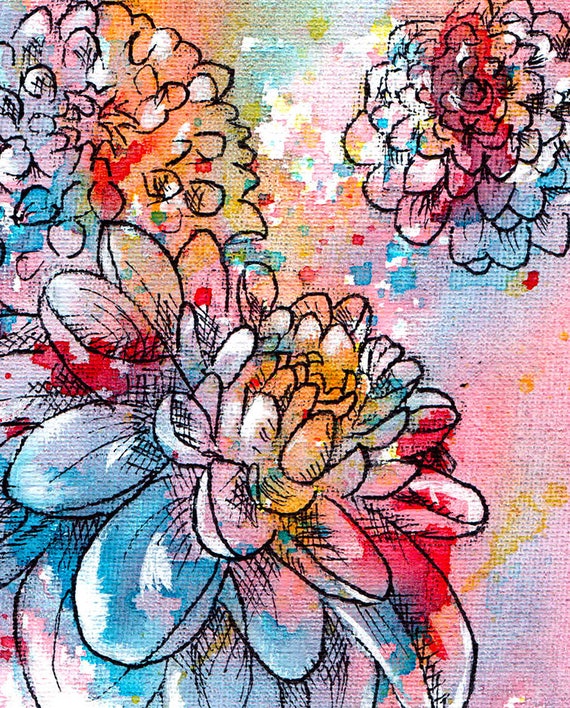This image is an artist’s rendition that combines elements of both painting and drawing, featuring three prominent flowers. The flowers are outlined in black, with splashes and splotches of various colors—reds, blues, yellows, pinks, oranges, greens, and whites—randomly applied throughout, giving the piece a vibrant and abstract quality. 

In the foreground, occupying most of the lower left area and extending toward the center, there is a large blooming flower with layers of petals that appear to wrap around in circles. This flower’s center is maroon, radiating out into hues of pink, blue, green, white, and turquoise. The middle section is a flurry of multicolored paint splashes, creating an energetic and lively visual effect. 

The upper right-hand corner features another medium-sized flower whose contours embrace the entire corner space, while the background itself reveals the texture of a canvas, with visible tiny lines. The overall composition suggests a dynamic interplay between structured outlines and the free-form application of watercolor, capturing the essence and spontaneity of floral beauty.